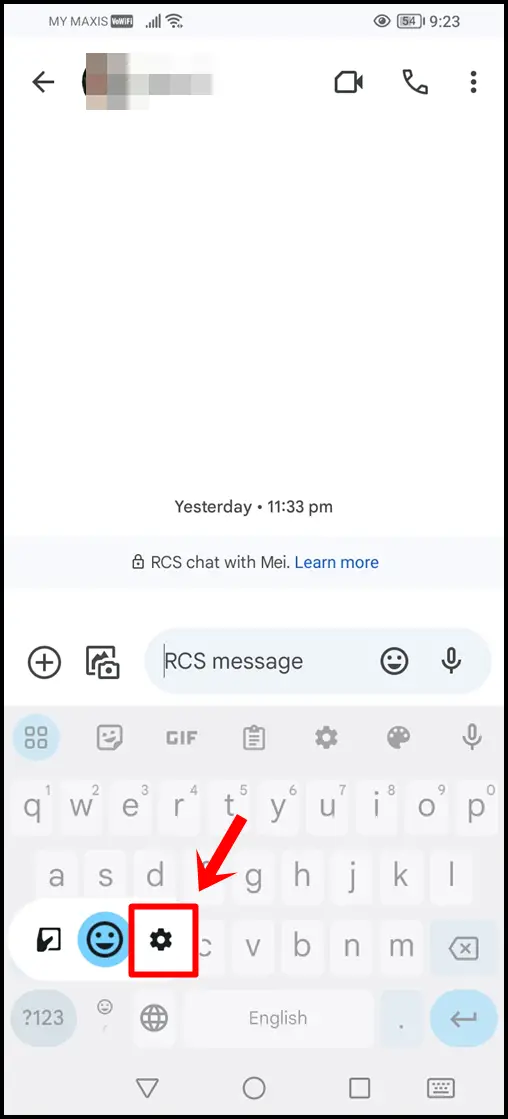The screenshot depicts a smartphone display enclosed by a thin black border. At the top of the screen, the words "My Maxis" are prominently displayed, with "MAXIS" spelled in uppercase letters. Adjacent to this, there are icons indicating the phone's cell signal strength, Wi-Fi connection, and battery life, which is at 54%. The time displayed is 9:23.

Just below this, the screen features a white background with a left-pointing arrow, followed by a pixelated, blurred-out image. To the right of this image are icons for a video camera, a telephone, and three vertically aligned dots.

In the midsection of the screen, the timestamp "Yesterday, 11:33 PM" is visible. Beneath this, a gray banner with a padlock icon and the uppercase text "RCS" is displayed. It is followed by the phrase "Chat with MEI," with "MEI" starting with a capital "M". The words "Learn more" appear in blue text next to this.

Further down, there is a circle containing a plus sign, a camera icon, and a text box that contains the words "RCS message." Adjacent to the text box is a circular icon with a smiley face, a microphone icon, and finally, a keyboard at the bottom of the screen. On the keyboard, a small gear icon is highlighted with a red box and an accompanying red arrow pointing to it.